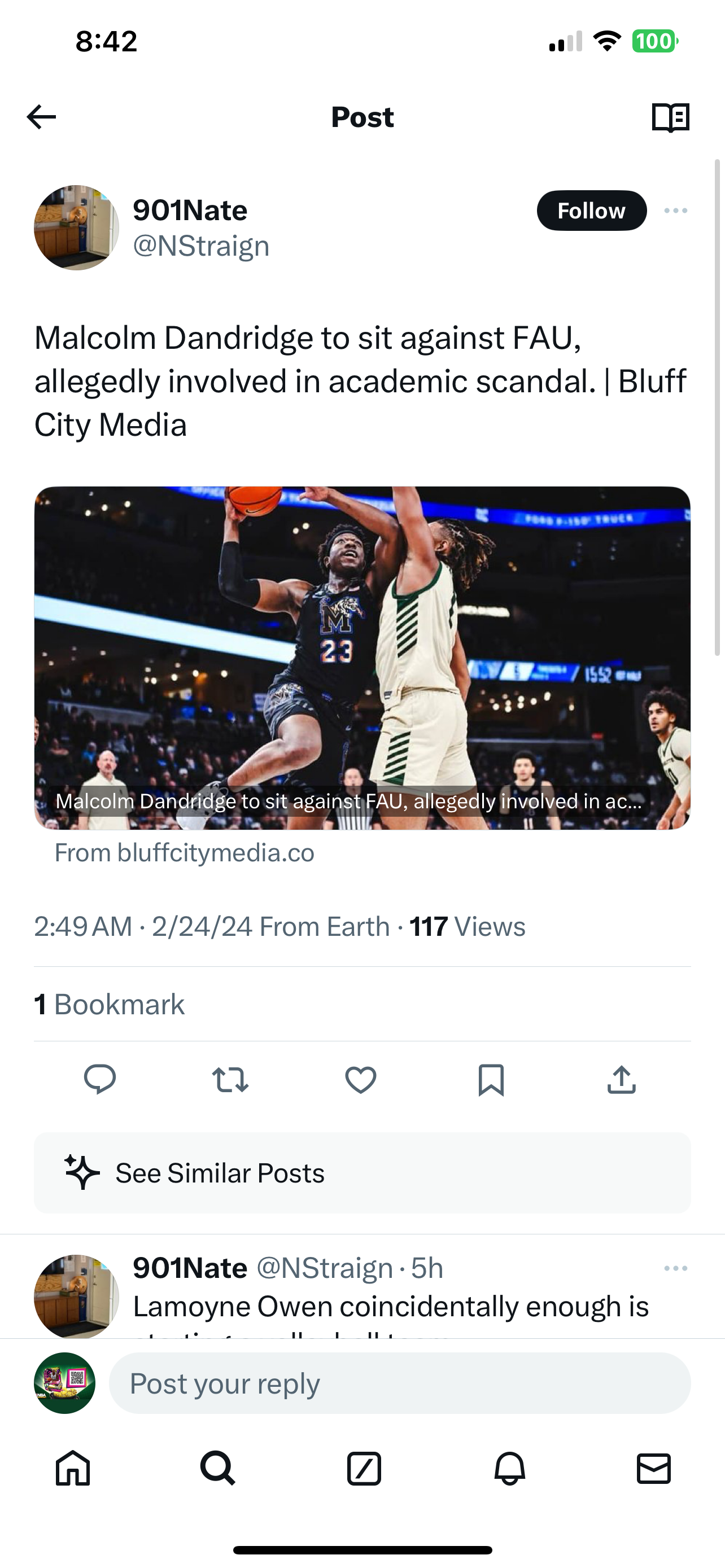The image displays a screenshot of a social media post found on a mobile phone. At the top of the post, in bold black text, it reads "POST". The post has been made by the user "901 Nate", whose handle is "@NSTRAIGN". To the right of the handle, there's a black button with the word "FOLLOW" written inside it, indicating an option to follow the user.

Below the user's handle, the post contains a headline that reads: "Malcolm Dandridge to sit against FAU, allegedly involved in academic scandal." This headline, attributed to Bluff City Media, suggests the involvement of Malcolm Dandridge in an unspecified academic scandal and his subsequent benching in a game against Florida Atlantic University (FAU).

Accompanying the headline is an image of Malcolm Dandridge himself, although the precise details of the image are not provided. Below this, there's a partially visible caption that starts with "LeMoyne Owen coincidentally enough is..." but the rest of the text is cut off and not discernible in the screenshot.